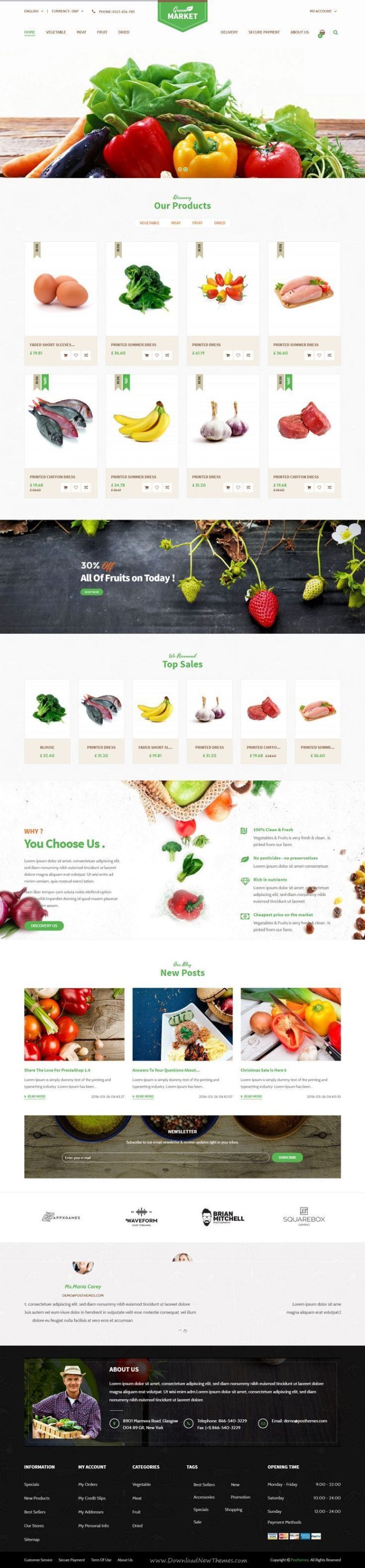In the slightly blurry, vertically-oriented image from a supermarket, a green logo with white text adorns the top center, its shape forming a triangle at the bottom center. Flanking the logo are words that likely list menu items. Directly beneath the logo is a horizontal image showcasing colorful produce, including peppers, a tomato, and assorted greens and carrots.

Below this are two rows of four small, vertically-aligned rectangular sections, each divided with a white background and tan bottom. Each section features a different type of fruit or vegetable. In the second row, identifiable items include bananas and garlic. These sections suggest purchasable goods.

Further down is another horizontal image displaying more fruits and vegetables against a black background, with identifiable items like a strawberry. However, the text accompanying the image is illegible.

Towards the bottom, another section exhibits various fruits and vegetables with additional informative text, though the blur makes it unreadable, limiting the amount of detailed information provided about this section.